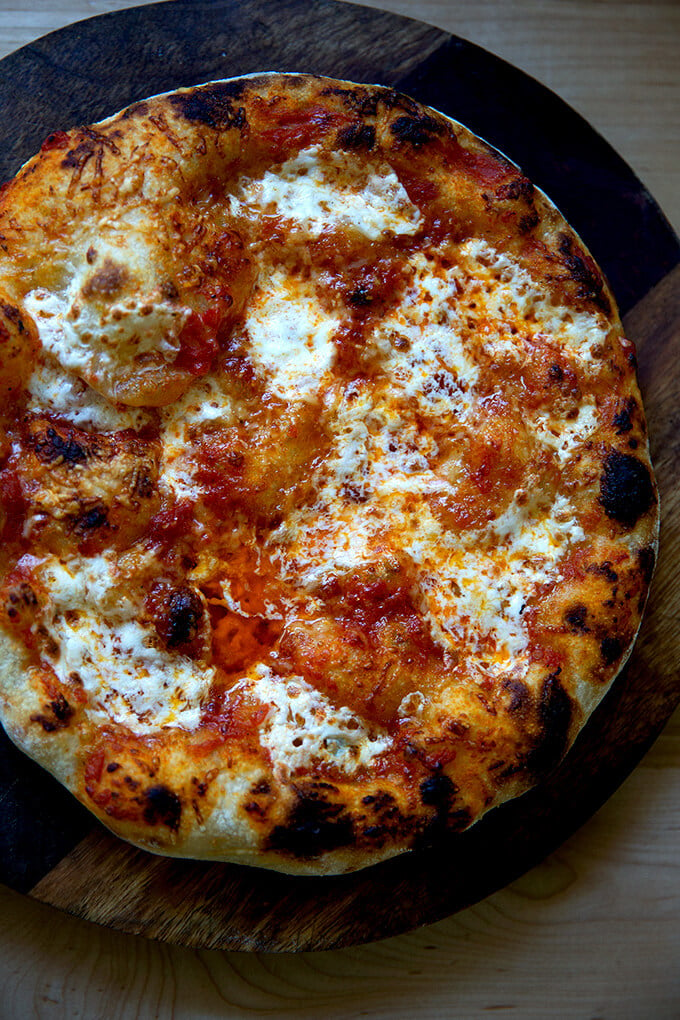A homemade pizza, captured in a vibrant and detailed photograph, occupies the frame in an upright rectangular portrait orientation. The pizza, which appears to have been baked in a high-temperature oven, sports a crust with tantalizingly crispy, almost blackened edges indicative of a traditional pizza oven. The irregularly shaped, hand-stretched crust reveals the artisan touch, far removed from the uniformity of a store-bought frozen pizza.

The surface of the pizza is adorned with a rich tomato sauce and a generous layer of melted cheese. The light source causes some glare, making it difficult to discern any additional toppings clearly, though the sauce bubbling up through the cheese suggests a perfectly executed bake. The cheese exhibits appealingly toasty spots, hinting at a delightful blend of textures and flavors.

This culinary creation rests atop a round wooden cutting board, which adds to the rustic, homemade aesthetic of the image. The cutting board itself is an interesting study in contrasts, with its segments displaying a gradient of wood tones. The top left portion is a medium shade, the center is almost black, and the bottom right transitions from a lighter color to a darker hue near a visible knot in the wood. This intricate backdrop enhances the overall presentation, making the pizza the focal point of a visually appealing and appetizing scene.